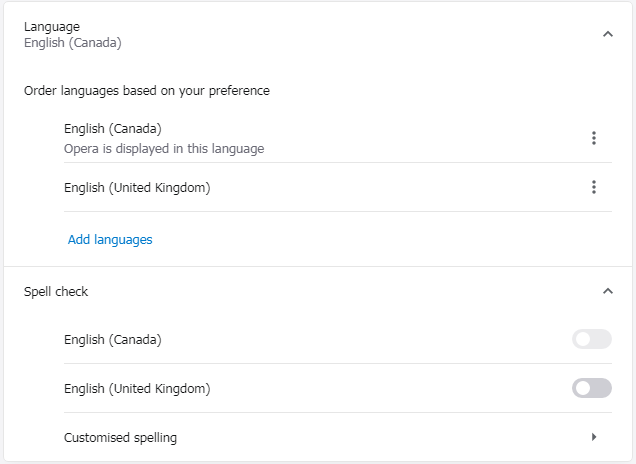The image depicts a language settings interface, likely from a web browser. The primary section displayed allows the user to configure their language preferences. Two languages are listed: "English (Canada)" and "English (United Kingdom)." Next to each language option are three vertical dots, suggesting additional settings for these languages. An instructional note indicates that the application (possibly Opera) is currently displayed in English (Canada). 

Below the language preferences is a spellcheck section with options for "English (Canada)," "English (United Kingdom)," and a "customized spelling" variant, where "customized" is uniquely spelled with an 'S' following British conventions.

Despite the clickable nature of these options, the viewer notes that clicking them yields no response. The interface likely offers further customizable settings if navigated correctly, suggesting that other categories or functions may be accessible by exploring additional menus or tabs. The screen mainly focuses on language and spellcheck preferences, providing users the ability to add new languages and adjust spellcheck settings specific to regional English variations.